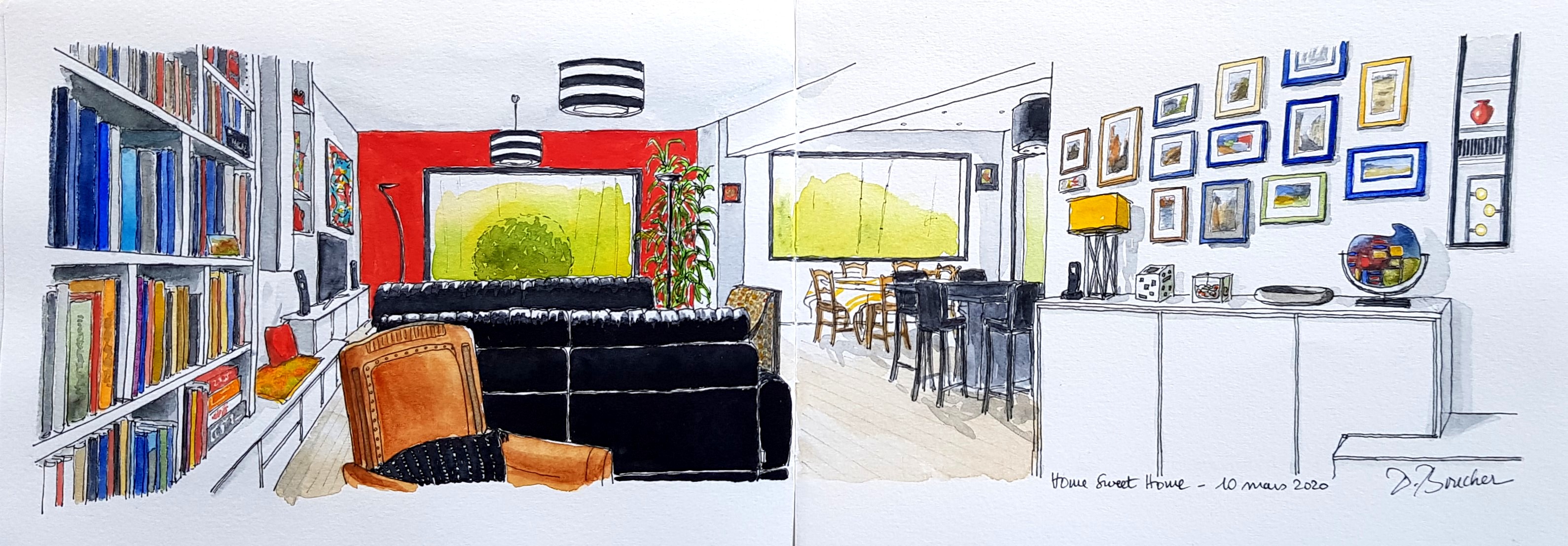This detailed drawing depicts a cozy living room scene. On the left-hand side, a tall bookcase brimming with books captures the viewer's attention. To the right of the bookcase, there is a large TV screen situated at the far end of the room. The right wall is adorned with numerous frames and albums, adding a personalized touch to the space. Below this display, a pristine white cabinet is prominently featured. The room is further brightened by a substantial window, contributing to the airy and inviting ambiance. Overall, the artwork thoughtfully illustrates a well-lived and comfortable living area.